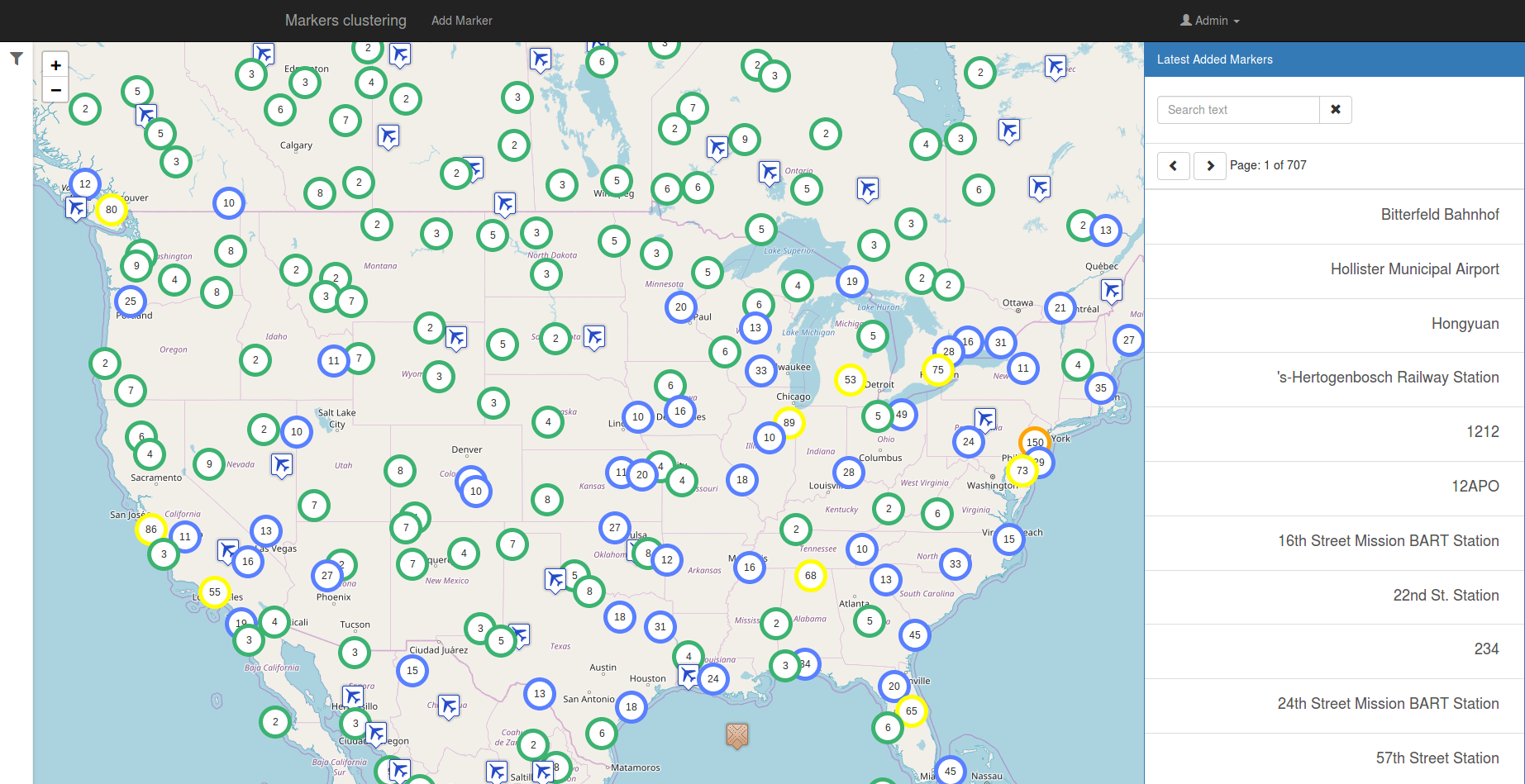In this image, we observe an interactive map interface filled with a variety of detailed elements. At the top of the map, a cluster of control buttons and options is prominently displayed. These include text labels and a tool for adding new markers to the map. The top right corner features an admin dropdown menu, which likely offers various administrative settings and tools. Below that, we see a display area highlighting the latest added markers, along with a search text bar for easy navigation.

The map itself is positioned on page 1 out of a total of 707, suggesting a vast array of data points. Key locations are cited with specific place names including Bitterfield, Bahnhof, Hollister Municipal Airport, Ungarn, Etelgenbosch Railway Station, 1212, 12th APO, 16th Street Mission Bath Station, 22nd Street Station, 234, 24th Street Mission Bath Station, and 57th Street Station. Additionally, broader geographical regions such as Arkansas, Austin, Houston, Denver, Nevada, Utah, Calgary, Montana, and Ontario are marked, indicating significant points of interest throughout these areas. The map provides a comprehensive and organized visualization of numerous locations, making it a valuable resource for detailed geographical analysis.